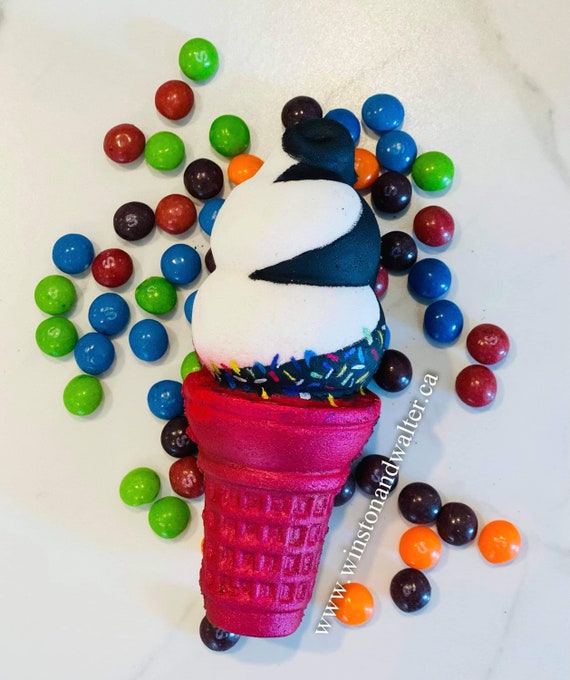This overhead photograph features a rubbery, purple ice cream cone with a squishy, faux ice cream scoop. The scoop is white and decorated with navy zigzag patterns and a speckled array of multicolored sprinkles. Surrounding the cone are various colored Skittles, including orange, red, green, blue, and black. A watermark in white text reads "www.winstonandwater.ca," suggesting an association with this website. Despite its realistic appearance, the entire setup exudes the texture and quality of a playful, squishy toy rather than an edible treat.